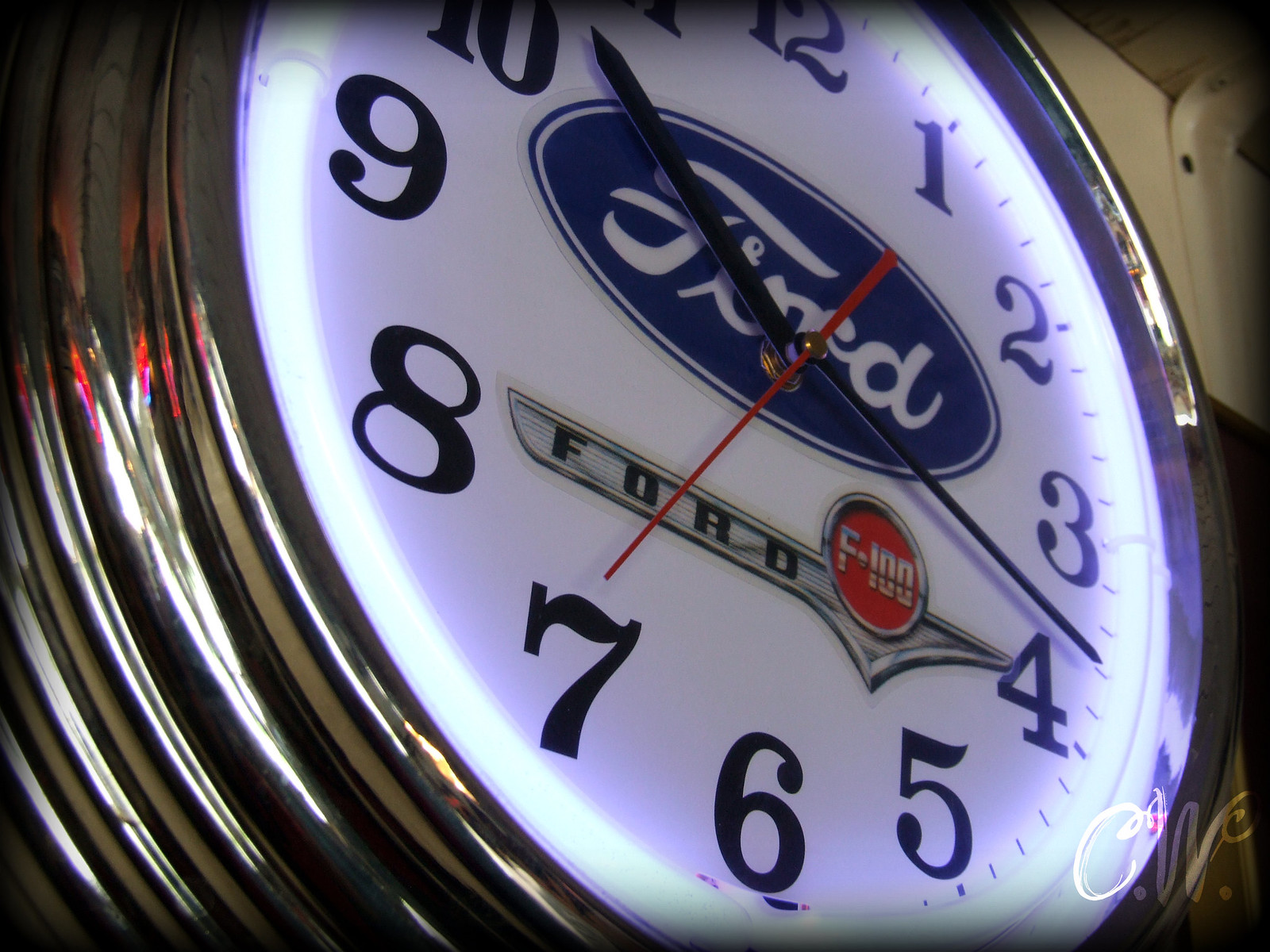This photograph captures a close-up view of a distinctive wall clock, which features a thick, chrome-style metallic frame resembling a car tire's rim. The clock's frame, polished to a mirror-like finish, is several inches thick, creating an impression of substantial depth. The reflective surface of the frame even catches a bit of light, possibly from a nearby window. The clock face is a bright, glowing white, bordered by a neon white light that adds a luminous halo effect around the edge.

The clock face displays bold black numbers from 1 to 12, with the current time showing the little hand on the 10, the big hand approaching the 4, and the red second hand crossing the 7. At the center of the clock face, the iconic blue Ford logo is prominently featured in an oval with white text. Below this, there is a red and silver F-100 Ford logo, adding to the automotive theme of the design. Additional details in the upper right-hand corner of the image hint at a cream-colored wall and bits of brown wood or metal, while a watermark "C.W." appears in the bottom right-hand corner.